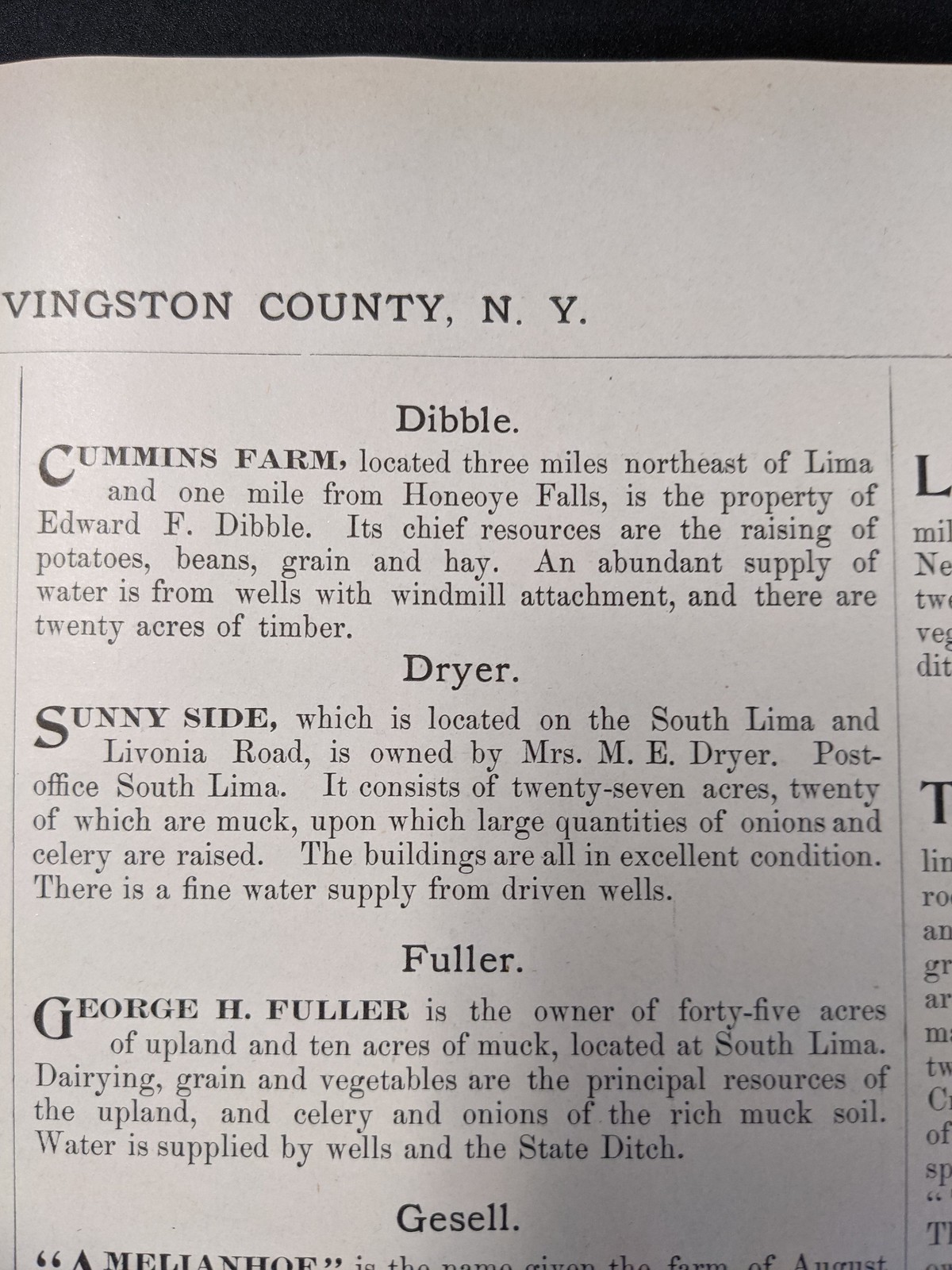The image depicts a vintage newspaper clipping showcasing property listings from Livingston County, New York. The top part of the clipping, featuring black text on a light grayish-white rectangular background, reads "Livingston County, N.Y." in all caps, although the 'L' and 'I' of "Livingston" are cut off. Below this header is a black-lined box divided into different sections, each detailing distinct properties.

The first listing concerns "Dibble Cummins Farm," located three miles northeast of Lima and one mile from Honeoye Falls, owned by Edward F. Dibble. This farm specializes in growing potatoes, beans, grain, and hay. It boasts an abundant water supply from wells equipped with windmill attachments and includes 20 acres of timber.

The second section highlights "Sunnyside Farm," associated with Mrs. Emmy Dreyer and situated on South Lima and Livonia Road. This property includes 27 acres, with 20 acres being fertile muck land ideal for cultivating onions and celery. The farm buildings are in excellent condition, with ample water provided by wells.

The final listing features George H. Fuller's farm in South Lima, which spans 45 acres of upland and 10 acres of muck. This farm produces dairy, grains, and vegetables on the upland soil, while the muck soil is primarily used for growing celery and onions. It also relies on wells and the state ditch for its water supply. 

To the right of the center column, some additional text from another column is visible but not completely readable due to being cut off.